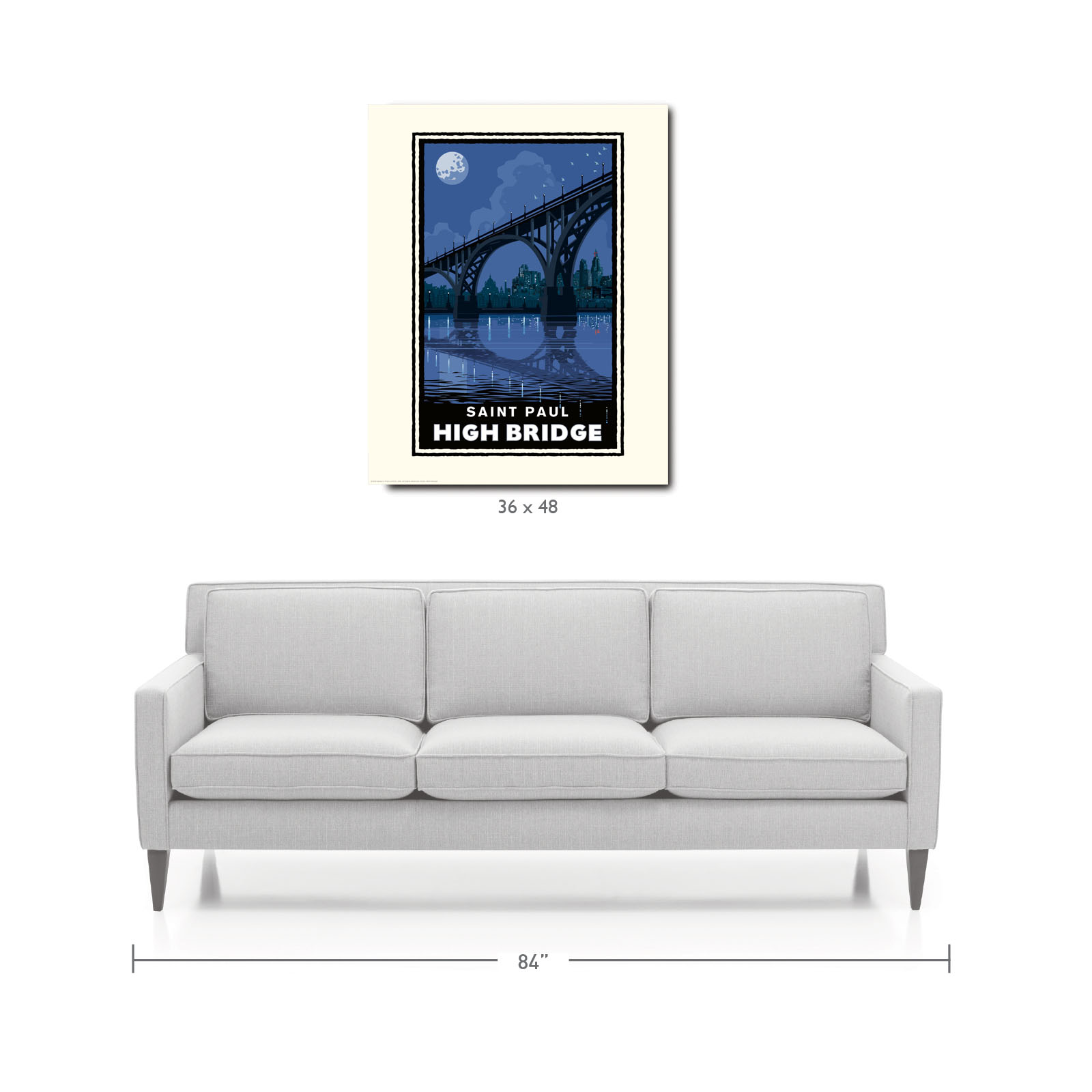This image is a minimalist advertisement showcasing a light gray, three-seater couch, and a piece of artwork on a plain white background. The couch, positioned at eye level, features armrests on either end and grayish-brown legs reminiscent of those found on a side table. It is 84 inches in length, clearly labeled beneath it. Above the couch, a framed picture of the St. Paul High Bridge is displayed. The artwork, measuring 36 by 48 inches, captures the bridge over a river at night, with the moon illuminating the scene in hues of blue, black, and gray. The bridge's name, "St. Paul High Bridge," is inscribed in white font at the bottom of the picture. The entire setup is shadowed for a more realistic effect, yet remains on a simple white background, emphasizing the furniture and the artwork's dimensions.